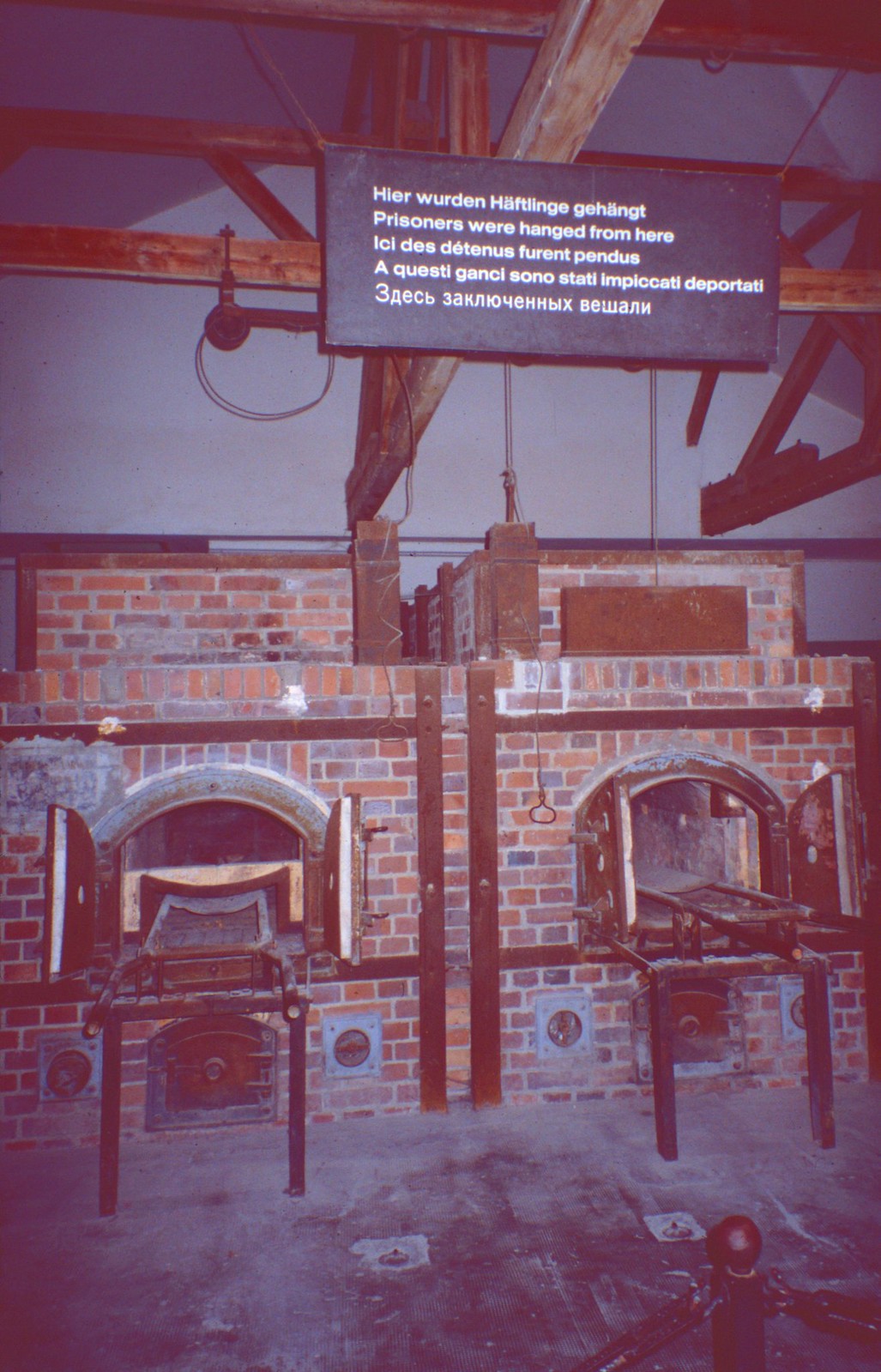This photograph depicts the grim interior of a World War II-era crematorium, likely associated with the Holocaust. The scene includes two red and clay brick ovens, designed for body incineration. Each oven features a contraption for sliding bodies in and out, and a compartment underneath for ash removal. The room has high ceilings supported by prominent wooden beams, from which ropes hang, accompanied by a large black sign written in five languages, including English, stating, "Prisoners were hanged from here." The dusty, dirty floor and a dark, somber atmosphere enhance the haunting and sobering nature of the site. The image appears to have an Instagram filter over it, suggesting it was shared on social media.